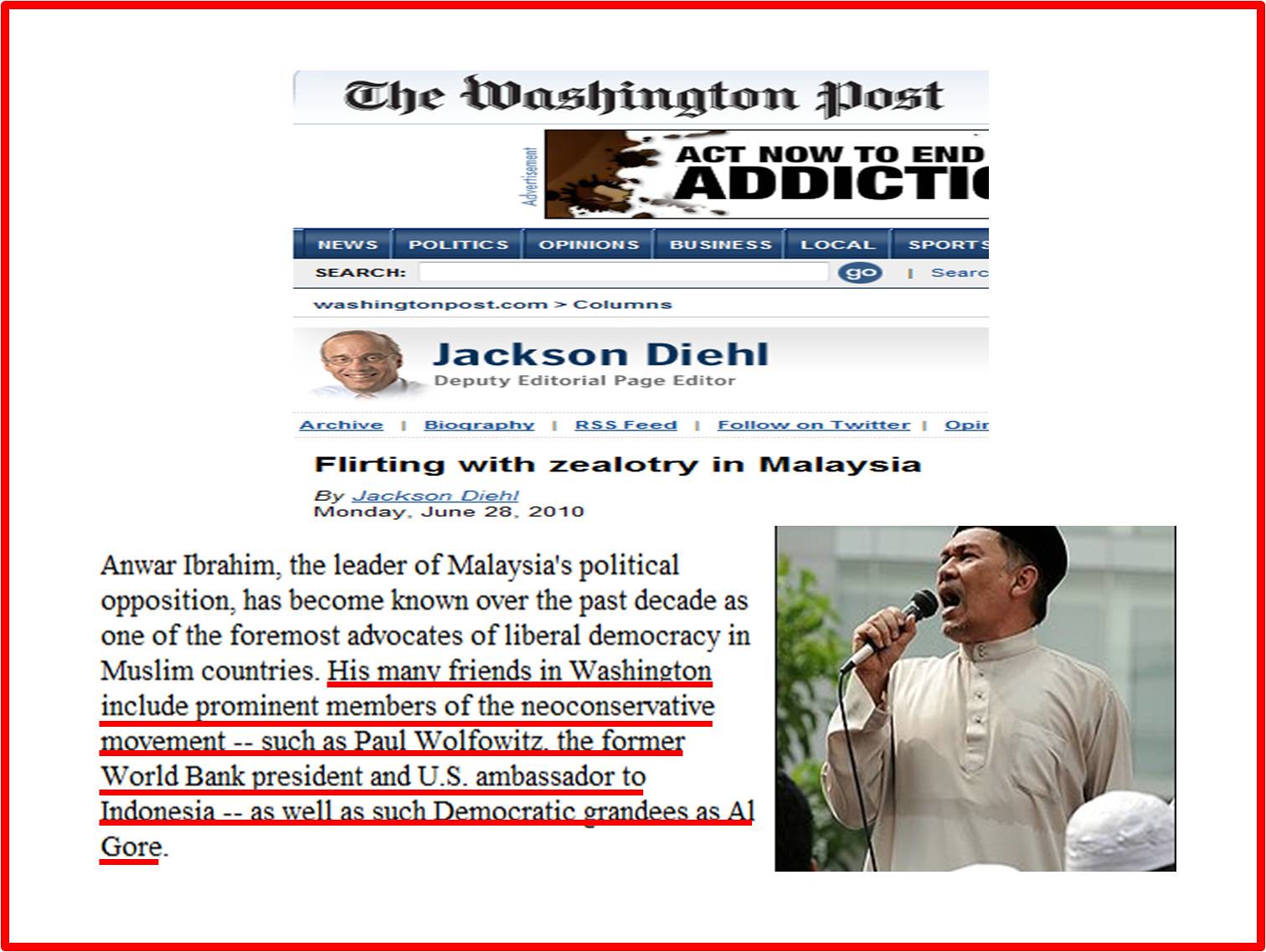The image is a screenshot of a Washington Post article with a white background and a red border. At the top, it prominently displays the Washington Post logo alongside an advertisement with the headline "Act Now to End Addiction." Below this, it shows a blue heading with the name "Jackson Diehl, Deputy Editorial Page Editor," followed by the article title in black, "Flirting with Zealotry in Malaysia by Jackson Diehl, Monday, June 28, 2010." The article highlights Anwar Ibrahim, the leader of Malaysia's political opposition, describing him as a key advocate for liberal democracy in Muslim countries over the past decade. A section of the text, underlined in red, mentions his many friends in Washington, including notable neoconservative figures like Paul Wolfowitz, and democratic grandees such as Al Gore. On the bottom right, there's a photograph of a man speaking into a microphone, likely Anwar Ibrahim. He is dressed in a basic off-white shirt with a mandarin collar and a black skullcap. Just visible in the lower right corner is the top of another person's white skullcap.